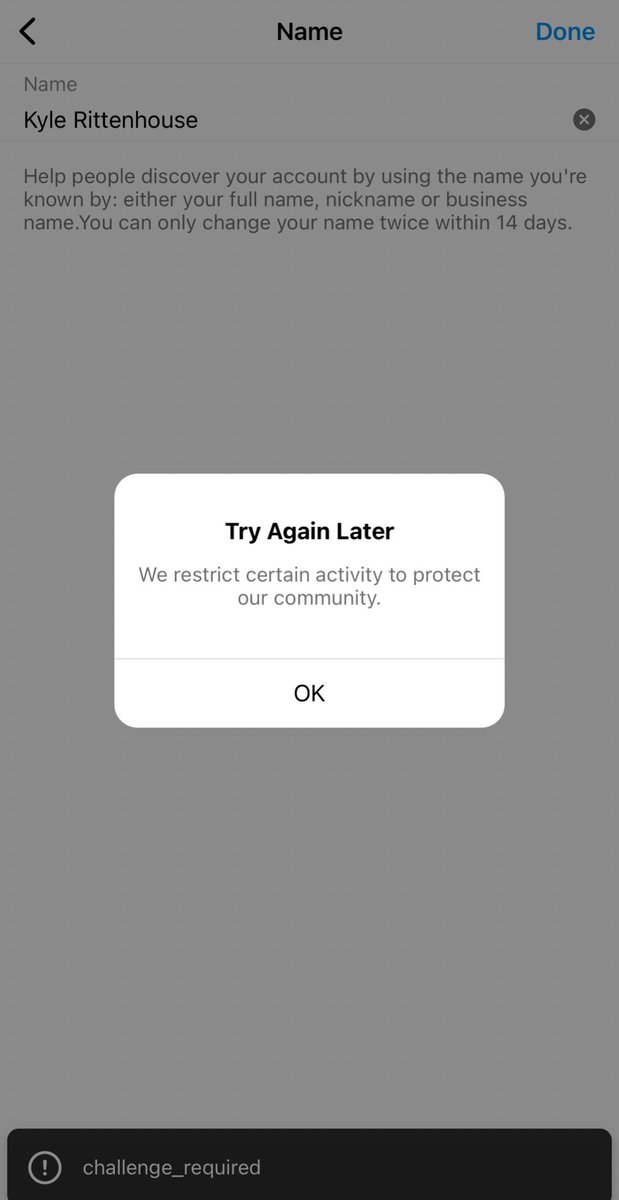The screenshot depicts a mobile interface with a predominantly dark gray background. At the center, a white, rounded-corner box appears with the message: "Try again later. We restrict certain activity to protect our community." Beneath this message is an "OK" button.

At the top of the screen, the interface includes a left-facing arrow labeled "Name," a blue "Done" button on the right, and an "X" to clear the text field. Below this, the text "Name: Kyle Rittenhouse" appears in black font, alongside a gray prompt: "Help people discover your account by using the name you're known by, either your full name, nickname, or business name. You can only change your name twice within 14 days."

At the very bottom is a black notification bar featuring an exclamation point within a circle, accompanied by "challenge_required."

Despite the gray background, all text remains legible, ensuring critical information is accessible.